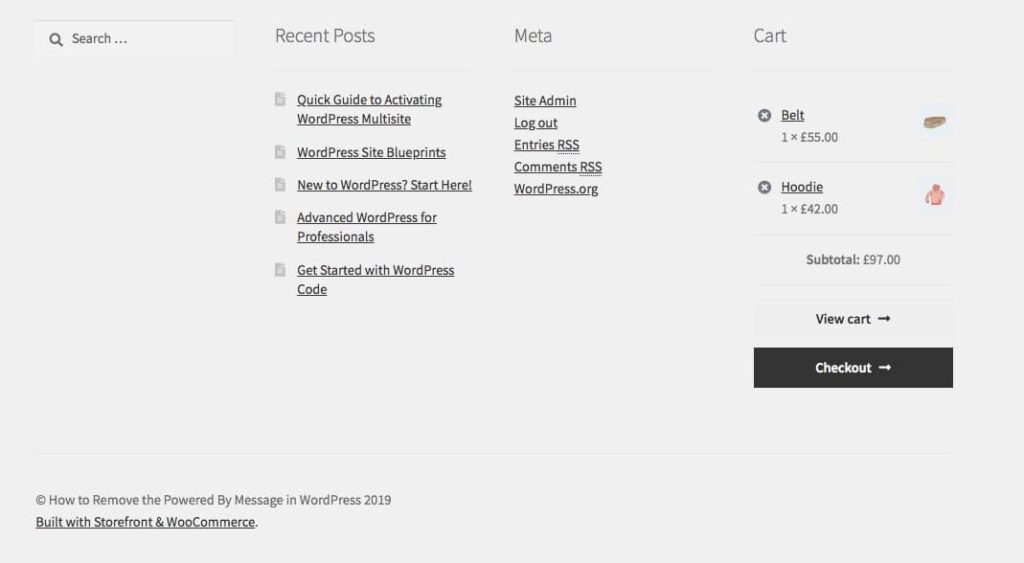**Detailed Descriptive Caption:**

This image is a screenshot of a section of a website with a layout consisting of four vertical columns on a light gray background. 

- **First Column:** At the top, a search bar is neatly integrated into the design, appearing recessed with a light-gray inner drop shadow effect. The search bar displays the word "Search" in black letters accompanied by a search icon on the left, hinting at its functionality.

- **Second Column:** Titled "Recent Posts," this section lists five links to different posts, each prefixed by a small document icon. The posts are:
  1. Quick Guide to Activating WordPress Multisite
  2. WordPress Site Blueprints
  3. New to WordPress? Start Here
  4. Advanced WordPress for Professionals
  5. Get Started with WordPress Code
  Each post title is presented in black text with underline, indicating they are clickable links.

- **Third Column:** Under the heading "Meta," this section includes five textual links:
  1. Site Admin
  2. Log Out
  3. Entries RSS
  4. Comments RSS
  5. WordPress.org

- **Fourth Column:** Labeled "Cart," this section displays two items in a shopping cart:
  1. **Belt:** Described as "1 x 55 euros," with an option to remove (indicated by an 'X' to the left) and a small image of a belt on the right.
  2. **Hoodie:** Listed as "1 x 42 euros," paired with an image of a pink hoodie, also positioned to the right.
  Below the item listings, centered text reports "Subtotal: 97.00 euros," followed by a thin gray line. Below this, “View Cart” is emphasized in bold with an arrow pointing right, and a black rectangle button at the bottom reads "Check Out" in white text with an arrow pointing right.

At the bottom left of the image, smaller text reads "Copyright: How to Remove the Powered By Message in WordPress 2019." Below this, a slightly darker and underlined link states "Built with Storefront & WooCommerce." 

This comprehensive breakdown encapsulates the structural and textual elements of the screenshot, offering a clear understanding of the webpage’s layout and content.